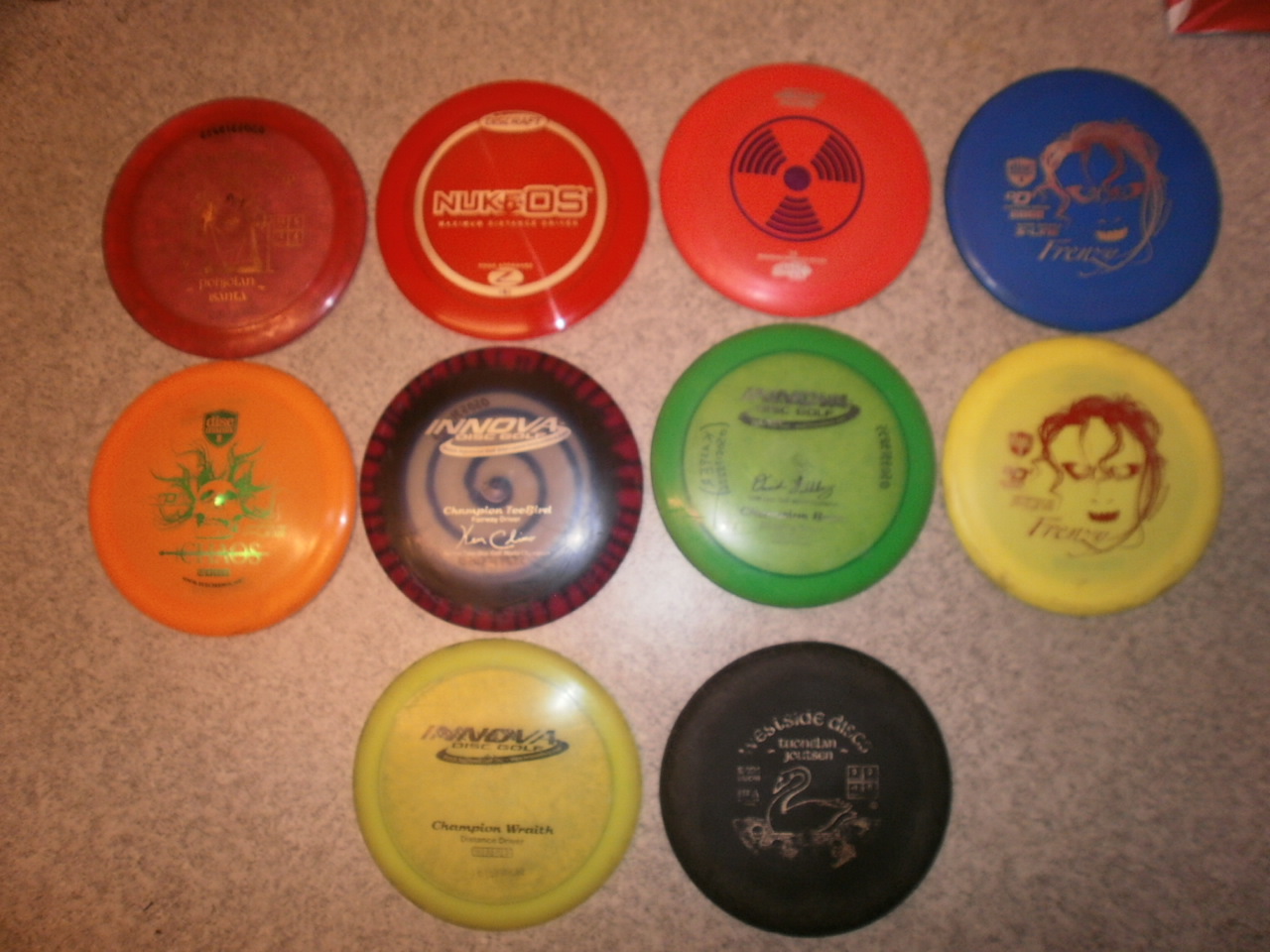This image showcases a collection of ten colorful frisbees arrayed on a speckled brown marble countertop. The frisbees are arranged in three neat rows: four on the top row, four in the middle, and two at the bottom. Each frisbee flaunts a unique design or logo in the center. The first frisbee in the top row is maroon, featuring a gold emblem and faded gold writing. Next to it, a red frisbee displays a golden circle encasing "NukeOS" in gold letters. A vibrant orange frisbee sports a smaller black circle with a radiation symbol, followed by another orange frisbee showcasing a gold-haired, gold-eyed, gold-mouthed face with the word "frenzy" faintly visible. Continuing the line, an orange frisbee is adorned with a green-outlined skull.

In the middle row, a maroon frisbee stands out with a black splotch, black spiral inside a gray circle, and white text reading "Inova" and "Champion Free Bird," along with a signature. Adjacent to it, a frisbee boasts maroon and black stripes blending into each other. The following lime green frisbee presents a subtle gradient to light green in the center, and another yellow frisbee showcases a face similar to the previous dark blue one but with red hair, red eyes, and the word "Frenzy." Lastly, a lime green frisbee spells out "Inova" and "Champion Wraith" in black text, while a black frisbee features a gold-painted swan and the words "Something Dreams."

These frisbees, in hues of red, blue, yellow, green, orange, and black, rest on a countertop that is described as tannish with gray streaks and specks of chocolate brown. Each frisbee is distinct, with some designs including a female face akin to a Frankenstein figure, a hazard logo, and various inscriptions.